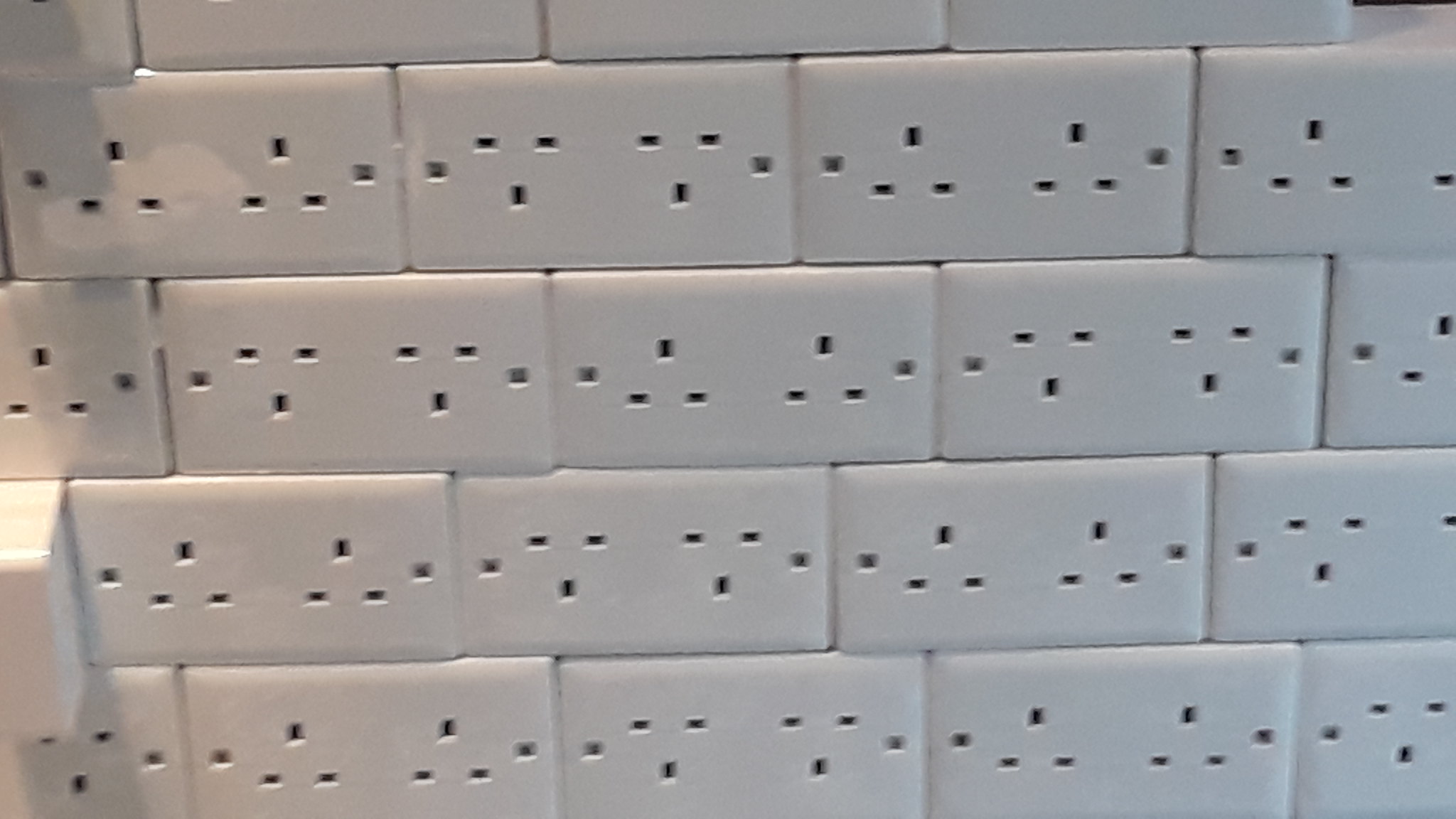The photograph depicts a wall tiled with numerous white blocks resembling electrical outlets. Each block features two receptacles arranged vertically, with the familiar three-pronged configuration for plugs. The blocks are arranged in a grid pattern, with the top row just partially visible due to the framing of the image. The outlet blocks vary slightly in orientation, with some appearing upside down. A total of eighteen blocks are clearly visible; most of them are neatly aligned, mimicking the appearance of stacked bricks. Uniquely, in the lower left-hand side of the image, one block appears to be protruding, creating the illusion that it has been pulled out from the wall. The pattern and the repetition of these outlet blocks create a striking, uniform visual effect across the wall.